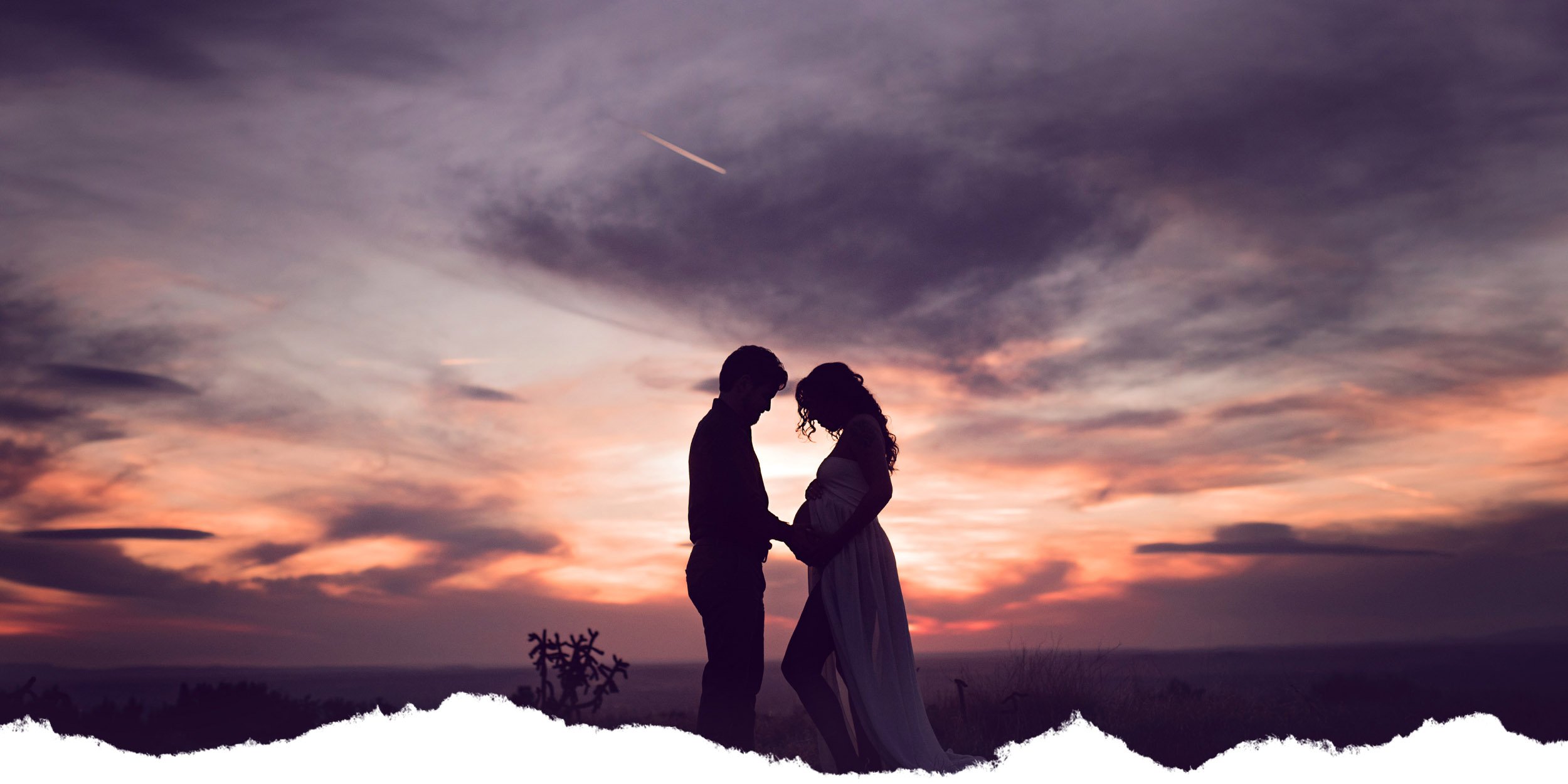This evocative photograph captures a tender moment during a vibrant sunset, with a rich sky painted in hues of purple, pink, and red. At the center of the image, a pregnant woman stands facing a man, their forms mostly silhouetted against the colorful evening sky. The woman's left leg is slightly bent, her long hair cascading over her shoulders, and she wears a flowing white dress that accentuates her serene appearance. The man, positioned on her left, gently places his hands on her belly, encapsulating an intimate connection between them. A jet's contrail, devoid of the visible plane, streaks across the sky, adding a subtle, dynamic element to the tranquil scene. The photograph has a jagged white edge at the bottom, suggesting an intentional crop that removes specific foreground details, leaving the focus on the couple and the mesmerizing backdrop. This small detail adds to the unique, almost dreamlike quality of the image.